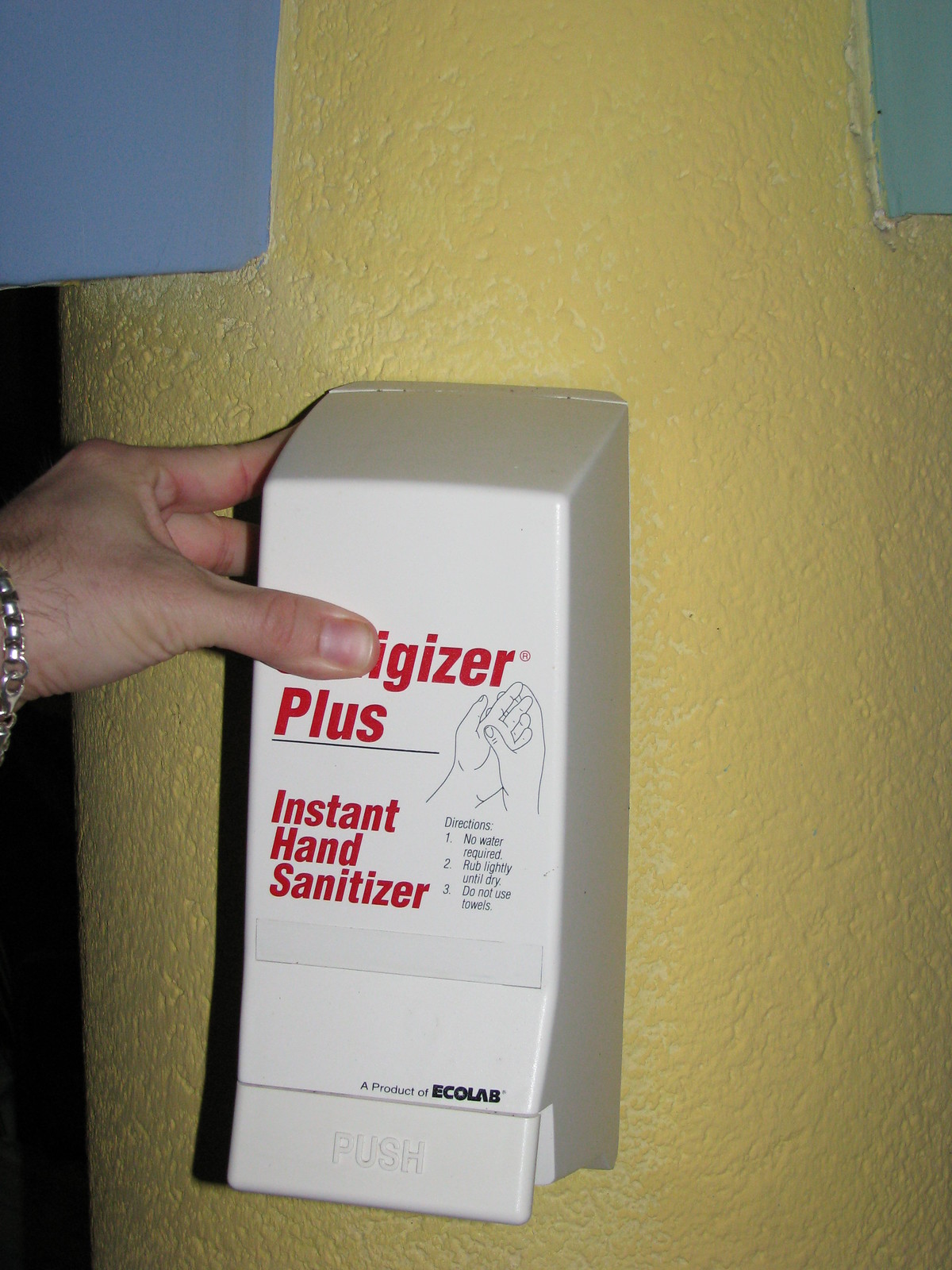The photograph is a close-up image of a white, rectangular hand sanitizer dispenser affixed to a bright yellow wall. The dispenser, a product of Ecolab, features raised text at the bottom that reads "PUSH." The container prominently displays an icon, illustrating the proper handwashing technique with two hands where the thumb of one wraps around the other hand. Directions printed in red on the dispenser state: "1. No water required, 2. Rub lightly until dry, 3. Do not use towels." Partially obscured by a hand on the left side of the image, the upper section of the dispenser also contains a label, potentially reading "EGIZA PLUS." The person positioned in the frame, identified as Kwakyeche, has their hand raised towards the dispenser, their thumb covering some of the lettering on the top line.